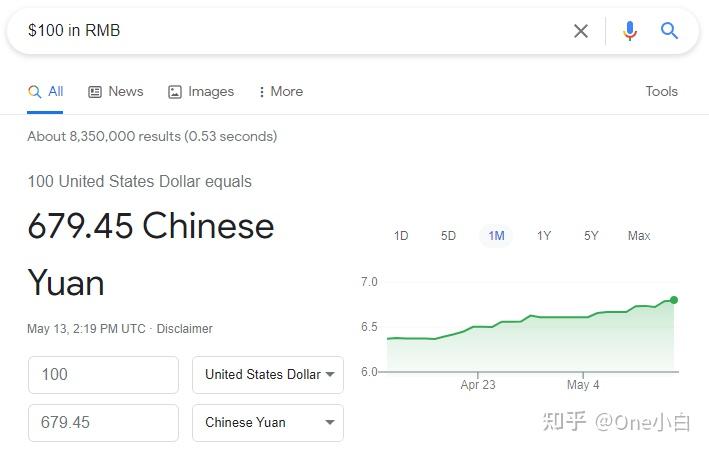The image showcases a detailed currency conversion between the United States Dollar (USD) and Chinese Yuan (CNY). At the top, a highlighted text box displays "$100 in RMB". Adjacent to this are options for "News", "Images", and "More". Beneath this, it shows that there are approximately 8,350,000 search results generated in 0.53 seconds.

The conversion rate is prominently displayed: "100 United States Dollar equals 679.45 Chinese Yuan". To the right, a green line graph illustrates the exchange rate trend from April 23rd to May 4th, depicting the Yuan's rise against the Dollar. The line on the graph is jagged, running from the left to the right.

A timestamp beneath the graph, labeled "May 13th at 2:19 PM UTC", is accompanied by a disclaimer. Another conversion rate is shown: "100 United States Dollar equals 679.45 Chinese Yuan", with a drop-down menu for currency conversions.

Below the graph, there are options to view different time intervals: "1 day", "5 days", "1 month", "1 year", "5 years", and "max". The current view is set to "1 month", explaining the displayed trend on the graph.